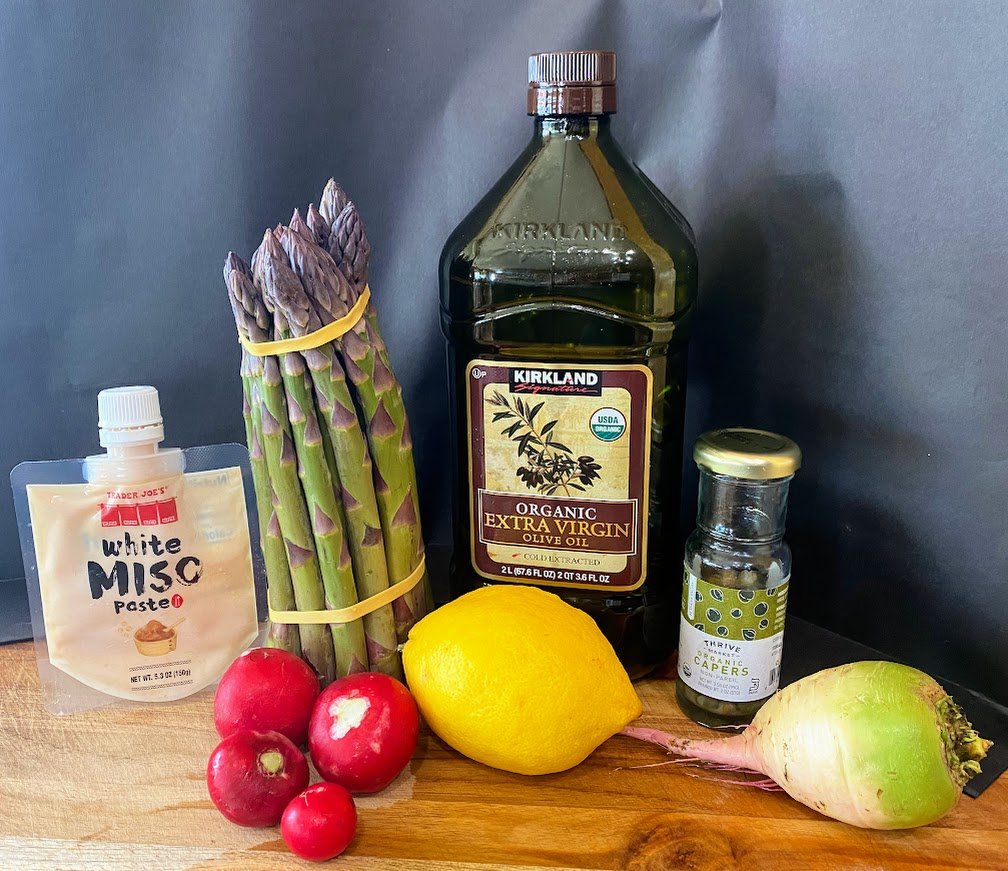This image displays a beautifully arranged assortment of ingredients on a wooden table set against a soft blue backdrop. Prominently featured on the left is a white miso paste from Trader Joe's, packaged in a squeeze tube with a yellow cap. Next to the paste is a bundle of fresh asparagus, bound together by two rubber bands, showcasing purple tips and vibrant green stalks. In front of the asparagus lies a quartet of red radishes, their colors contrasting nicely with the green vegetables. Central to the composition is a tall bottle of Kirkland Organic Extra Virgin Olive Oil, adorned with an illustration of an olive branch and the USDA organic seal. Just below this bottle sits a bright yellow lemon. To the right, there is a smaller bottle of capers with a bronze-colored twist-off cap. Finally, to the far right, rests what appears to be a turnip or parsnip, with its light green top fading into yellow and transitioning to a pinkish hue at the root. The arrangement and variety of ingredients suggest the preparation of a delightful meal, reflecting a touch of Mediterranean cuisine.